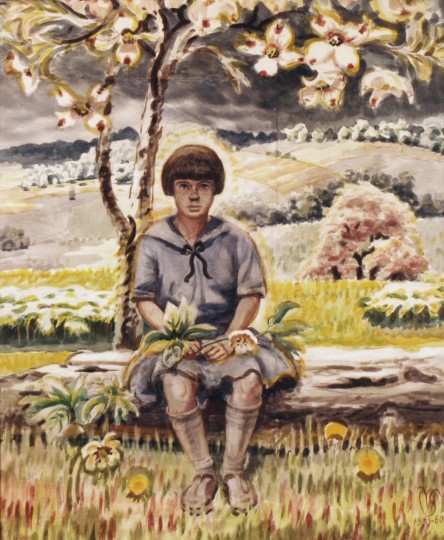This image showcases a beautifully detailed painting of a young girl sitting on a log in an outdoor setting. She has short brown hair with bangs and is dressed in a light blue dress that reaches her knees, adorned with a small collar and a bow at the neck. She wears knee-high white or cream-colored socks along with tan shoes. The girl, positioned centrally in the image, is holding a yellow flower, possibly a large lily, in her hands, while surrounded by a field of wildflowers in various shades of white and yellow. 

Behind her, a magnificent flowering magnolia tree in full bloom displays white blossoms with red tips. The background unfolds into rolling hills dotted with more white flowers and pink flowering trees, under a moody, gray marbled sky. The painting employs an impressionist style, with brush strokes that blend softly to create a dreamlike, slightly blurred effect, enhancing the serene and picturesque quality of the landscape.